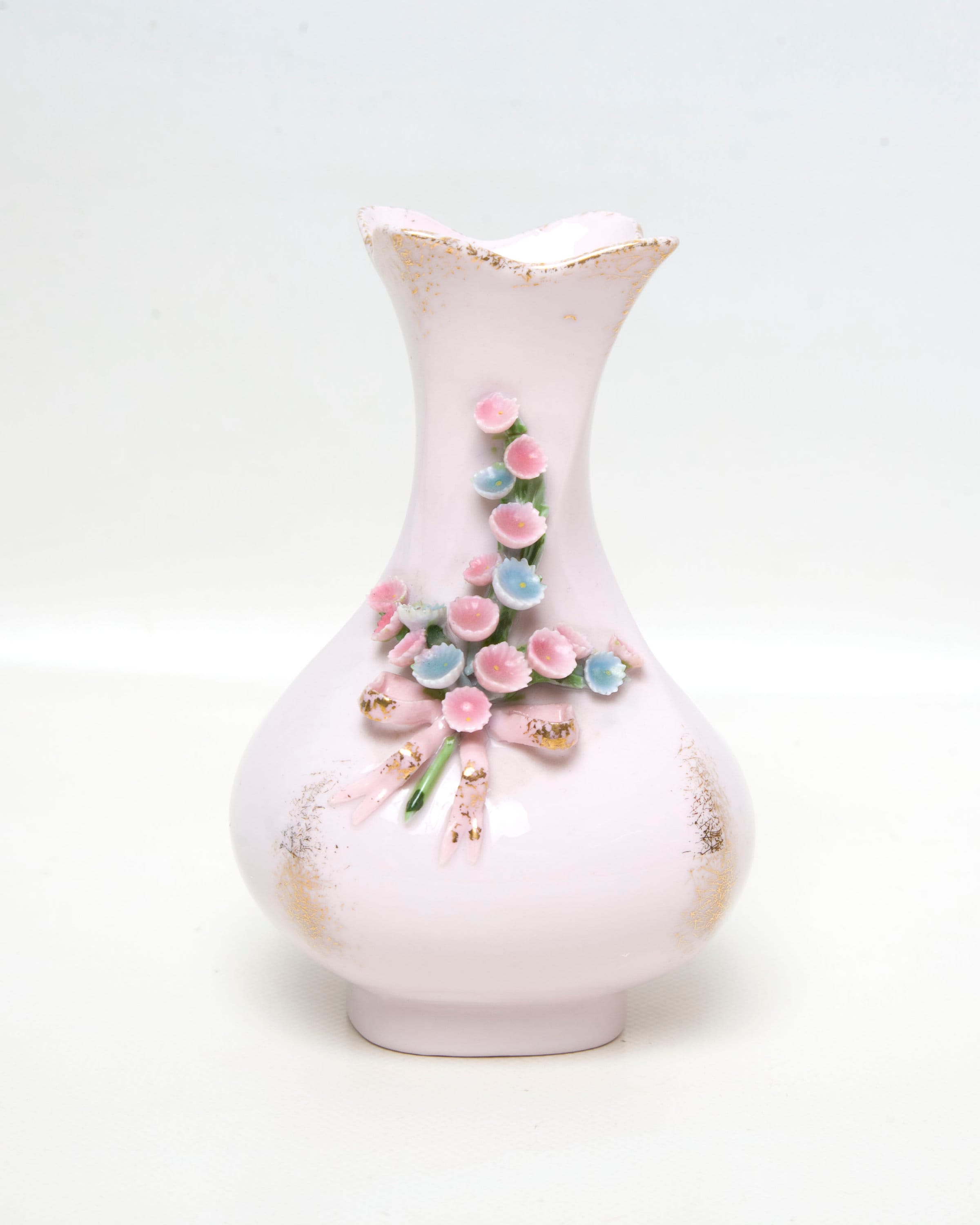This photograph features a vintage, white porcelain vase with an aged patina. The vase exhibits various orange and brown discolorations, indicative of its antiquated nature. Toward the center, it is adorned with delicate floral details, showcasing intricately painted white and pink blossoms accompanied by soft blue flowers. These florals are connected by a solitary green stem that trails towards the base of the vase. The vase is positioned on a pristine white surface, which is set against a similarly white background. Subtle shadows cast by the vase create a sense of depth, while the faint pink backdrop near the green stem adds a touch of color. Additionally, traces of orangey and brown dirt are noticeable in this area. The vase captures and reflects light, accentuating its timeless elegance.